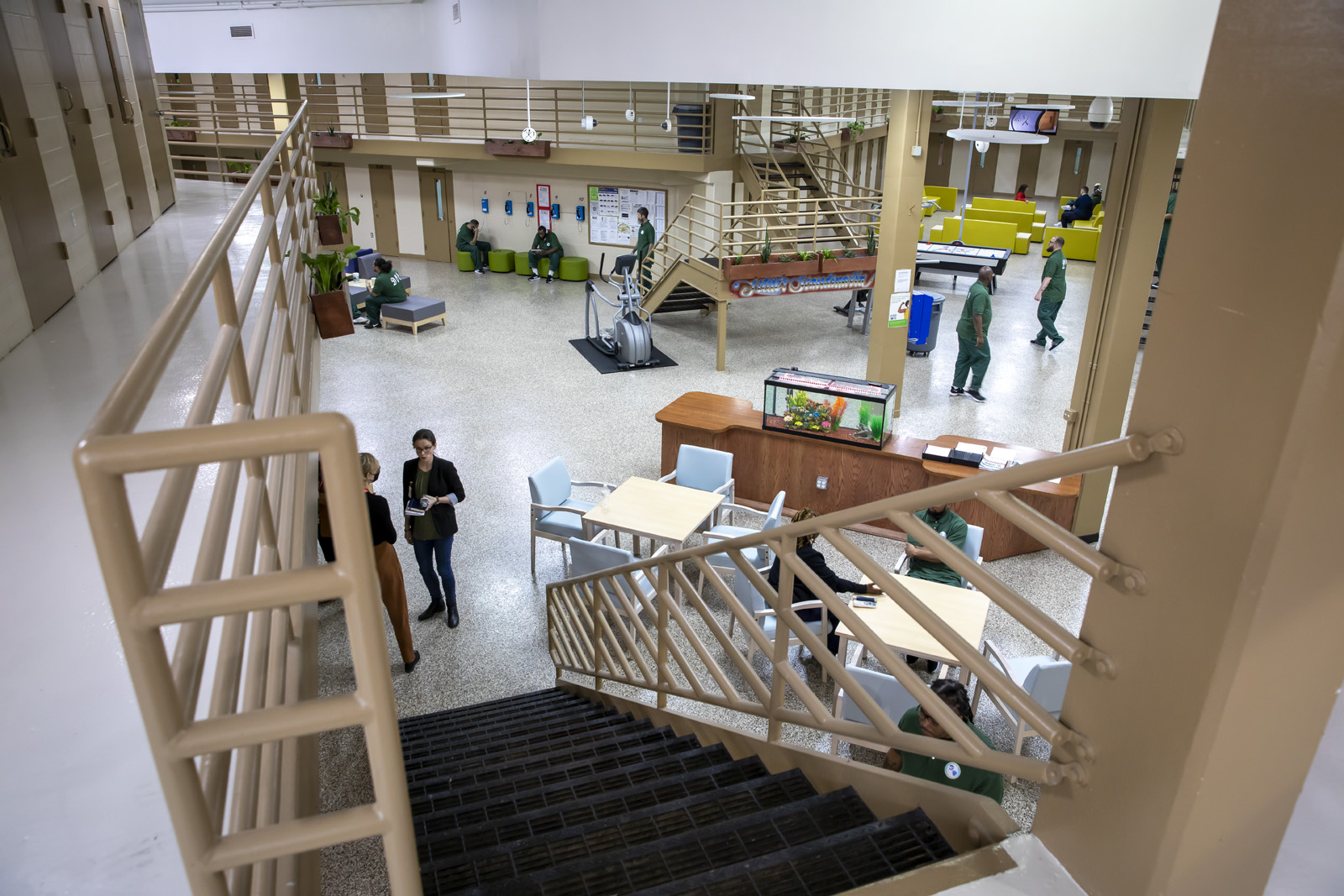The photograph showcases a well-organized, multi-level correctional facility resembling a social or recreational area within a prison. The upper level features beige and brown striped walls with light brown metal railings, and white linoleum floors. A key feature of this upper level is a staircase with brown steps leading down to the lower level. At the bottom of the staircase, two women, one facing away and the other facing the camera, stand in what appears to be business attire. 

The lower level includes various recreational and functional areas: a recognizable small social space with blue chairs around a table, a brown piece of furniture holding an aquarium, an exercise area with an elliptical machine on a black mat, and numerous lime green couches clustered around a television. Additionally, there are two people seated near some payphones and multiple individuals wearing green uniforms resembling scrubs, possibly inmates, dispersed throughout the scene. The entire environment exudes a clinical and orderly atmosphere, characteristic of a jail or correctional facility.